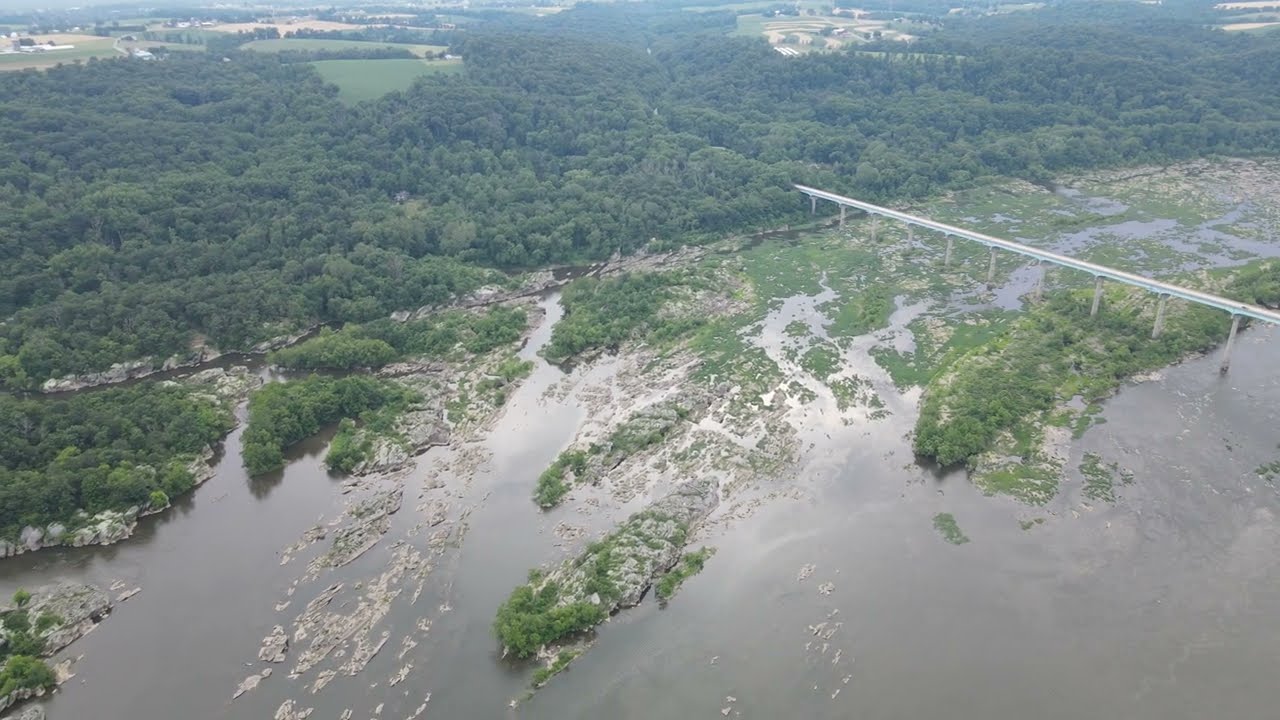This aerial photograph, taken during the daytime with a slightly foggy ambiance, captures a detailed and expansive view of a wide body of water that spans from the lower corners towards the center of the image. The water, which could be a river or possibly a lake, is somewhat flat and gives an impression of being shallow, interspersed with numerous small, rocky and grassy sandbars. A notable feature of the scene is a tall, narrow bridge crossing the water diagonally from the upper left to the upper right, supported by ten vertical columns. This bridge connects various parts of the landscape. Surrounding the water, especially near the shoreline, a dense forest of tall green trees stretches out, eventually giving way to farmland and small towns visible in the upper part of the photograph. The overall view suggests a serene, natural setting with no visible human activity, taken from a high vantage point, possibly by a drone. The photograph resembles a high-definition television screen in shape.